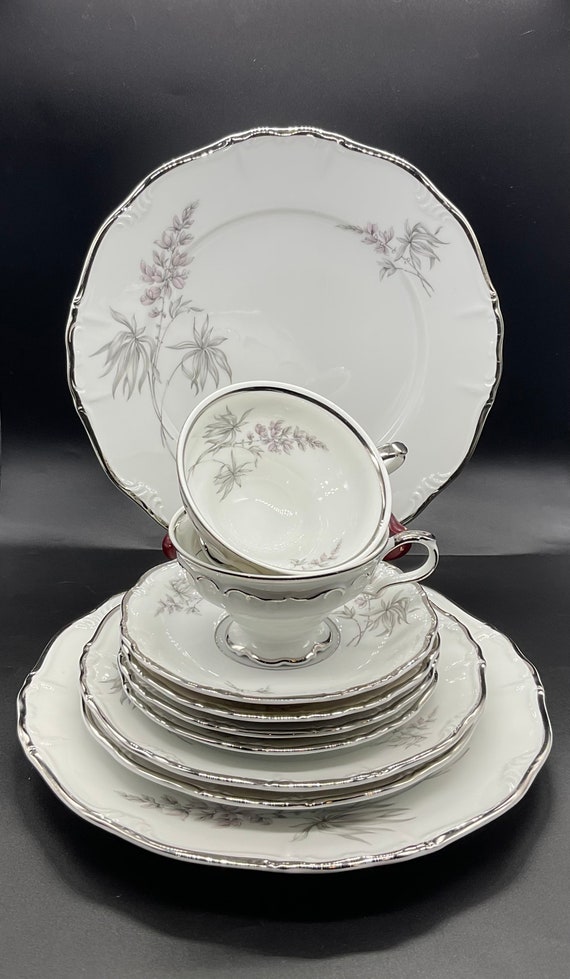This color photograph showcases a meticulously arranged set of vintage fine china dinnerware, featuring a prominent large round plate positioned upright at the top of the image. Below it, a tiered stack of glossy, white plates adorned with delicate, dainty floral patterns depicting grayish branches with clusters of small pink flowers catches the eye. The plates, arranged in ascending order of size, transition from dinner plates to saucers, and finally to two elegant teacups. One teacup is placed neatly on a saucer, while the other rests diagonally above it, highlighting their thin, refined structure. The background is a dark gray, which provides a stark contrast and enhances the shine of the fired or glazed exterior of the crockery, accentuating its sophisticated and charming appearance.